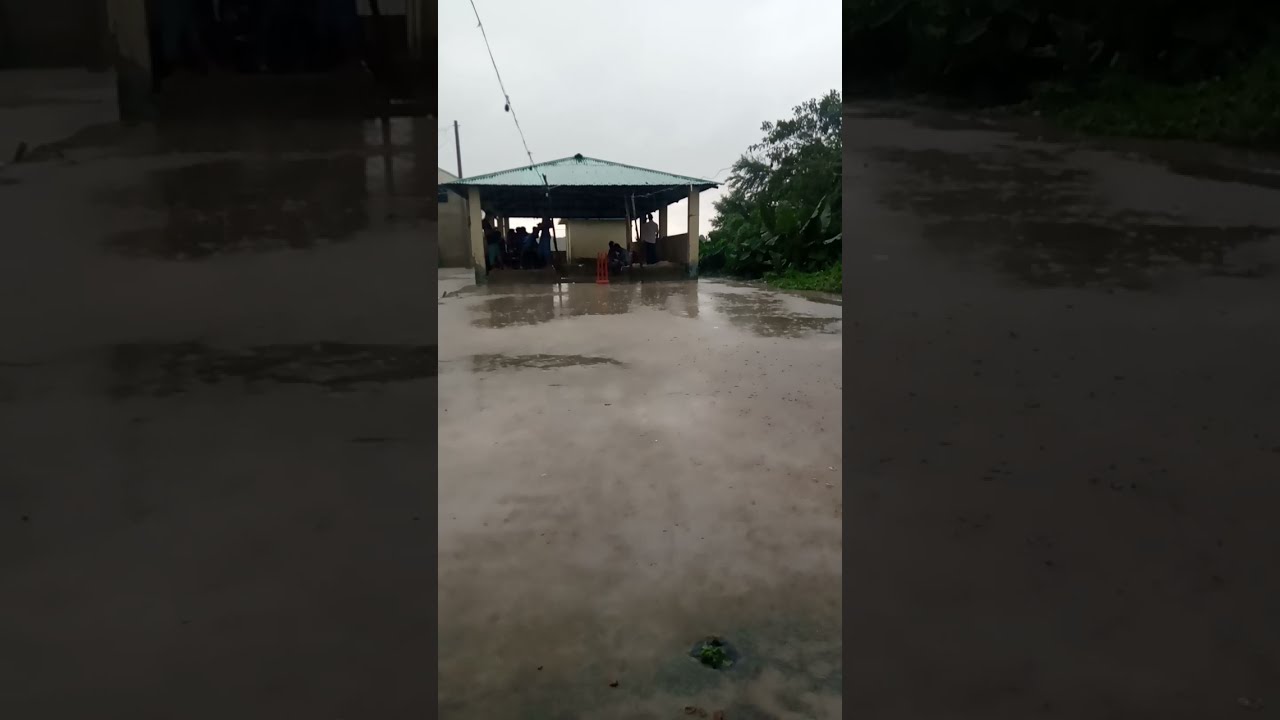The image depicts a rainy scene centered around a wet, expansive concrete surface that dominates the foreground, gleaming under the gray, overcast sky. In the background stands an open-air shelter with a distinctive green pyramidal roof supported by white posts at each corner, giving it a pavilion or hut-like appearance. The shelter contains some indistinct objects, possibly boxes or a cubic structure, and seems to have at least one person standing and another sitting under its cover. White, low half-walls line part of the shelter on the right, adding to its structural complexity. Flanking the shelter are green trees with small leaves, providing a natural contrast to the man-made environment. To the left of this central structure, part of another building can be seen, with a wire—likely for power or lighting—stretching from above the camera's vantage point to the shelter. The overall photograph, which appears somewhat dark due to the stormy weather, is bordered by two vertical bars on either side, providing zoomed-in views of the main image, emphasizing the wet and rainy conditions of the scene.